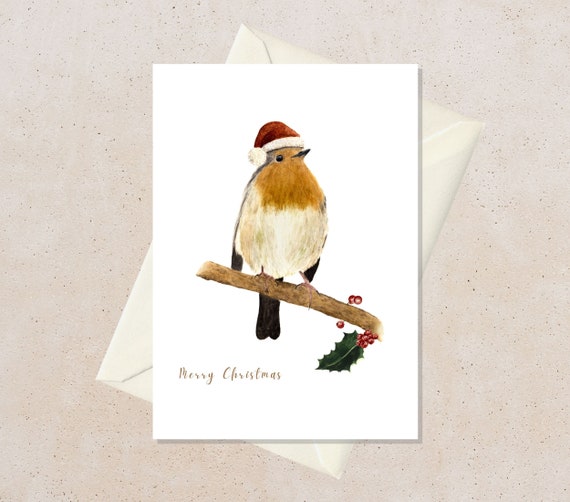The image features a Christmas greeting card set against a square-sized, beige background with subtle pockmarks. The closed card showcases a whimsical bird wearing a red and white Santa hat, perched on a tree branch adorned with a single green holly leaf and small red berries. The bird has a black tail, a black beak, and black eyes, with distinctive coloring that includes an orange chest, black feathers around its neck, and a whitish stomach with hints of brown. In the bottom left corner of the card, the phrase "Merry Christmas" is elegantly inscribed in gold letters. Accompanying the card, a backwards-placed envelope sits behind it, displaying an off-white color. This entire setup rests on a slightly textured, manila-like surface.